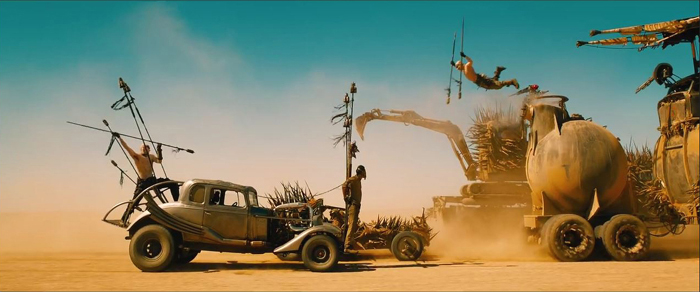In this detailed scene from the movie "Mad Max: Fury Road," an intense, post-apocalyptic chase unfolds in the desert under a clear blue sky. Several heavily modified, makeshift vehicles are involved in a ferocious battle. On the right side, a jeep-like vehicle commandeered by two individuals armed with spears is visible. One warrior stands at the front and another at the back, poised for combat. Amid this chaos, a man is seen leaping through the air with a spear in each hand, seemingly descending from a mechanized "horse car," a vehicle modified to resemble a primitive horse carriage but powered by an engine.

In the center of the image, a 1932 Ford-style car is prominently featured; this iconic car is where Mad Max is famously strapped. Pursuing this car is a massive semi-truck towing a large, multi-gallon trailer filled with milk, which is being targeted for attack. On top of the trailer, a man is captured in the act of jumping off, armed with explosive devices, ready to sabotage the pursuing vehicles. Among the attacking convoy, there are also larger vehicles such as a makeshift cement mixer and a tractor, adorned with spikes and spears, all hurtling through the sandy landscape in this captivating and dynamic cinematic moment.